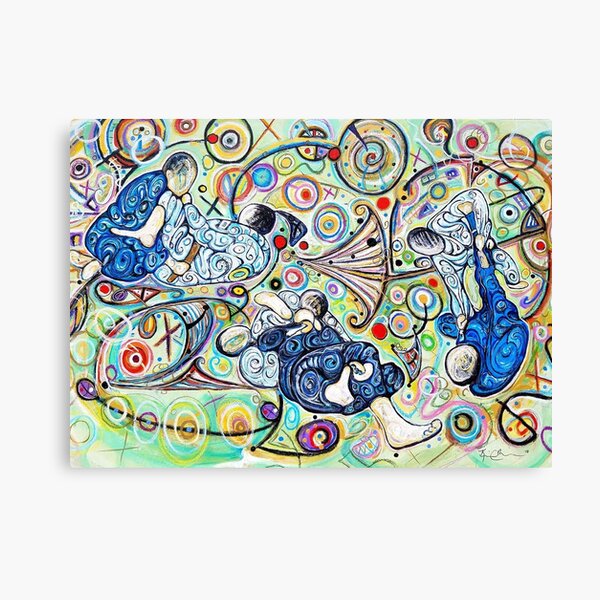This vivid abstract painting, set on a white canvas and hung on a plain white wall, prominently features three sets of figures that appear to be sumo wrestlers or individuals practicing karate. The characters, depicted in dark blue and very light blue robes, engage in various martial arts poses, suggestive of combat. Dominating the foreground is a pronounced foot of one figure in dark blue. The background is teeming with an array of vibrant colors—red, yellow, orange, green, blue, purple, black—forming an intricate mosaic of shapes, including circles and X’s, evoking a fantastical mix of Picasso and Dali's stylistic elements. The scene portrays the figures interacting against a backdrop rich in hues, adding depth and intensity to the overall composition.